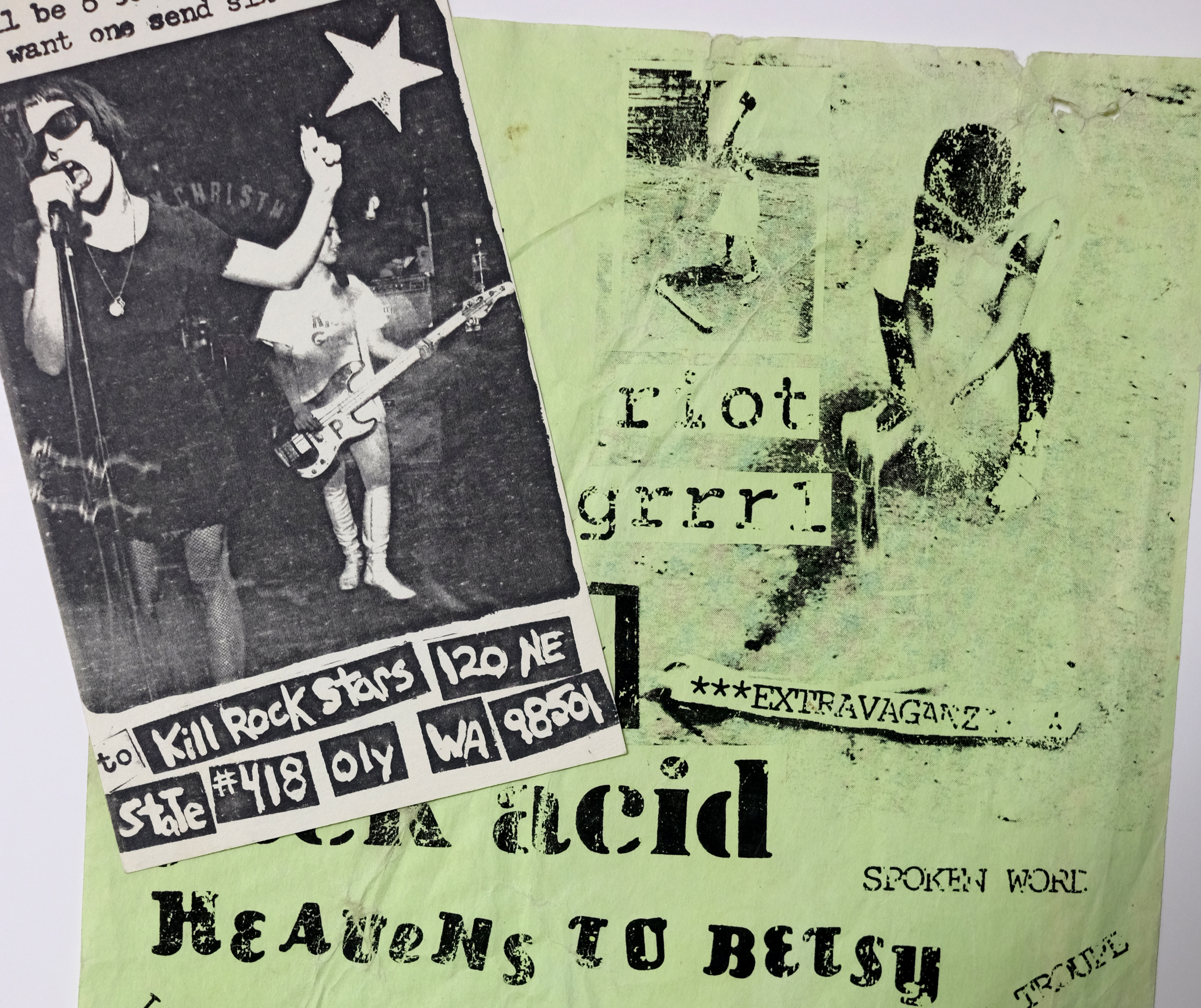This square-shaped image, approximately 5 inches by 5 inches, features two overlapping pieces of paper. The top paper is a slightly angled, black-and-white, faded, xeroxed clipping of an old newspaper. Dominating this clipping is a grainy photograph of two women: one in a black dress wearing sunglasses, holding a microphone and singing, and another in the background playing a guitar and dressed in white, near a white star in the corner. Below the image, text reads, "Kill Rock Stars, 120 N.E. State, No. 418, Oly, Washington, 98501."

Beneath this newspaper clipping is a faded, light green piece of paper. Though heavily worn and difficult to decipher, visible text includes the words: "Riot Grrrl," "Extravaganza," "Acid," "Heavens to Betsy," "Spoken Word," and "Troop," each appearing in various fonts and sizes. The background shows faint, indiscernible images and letters, adding to the vintage and distressed aesthetic of the entire composition.